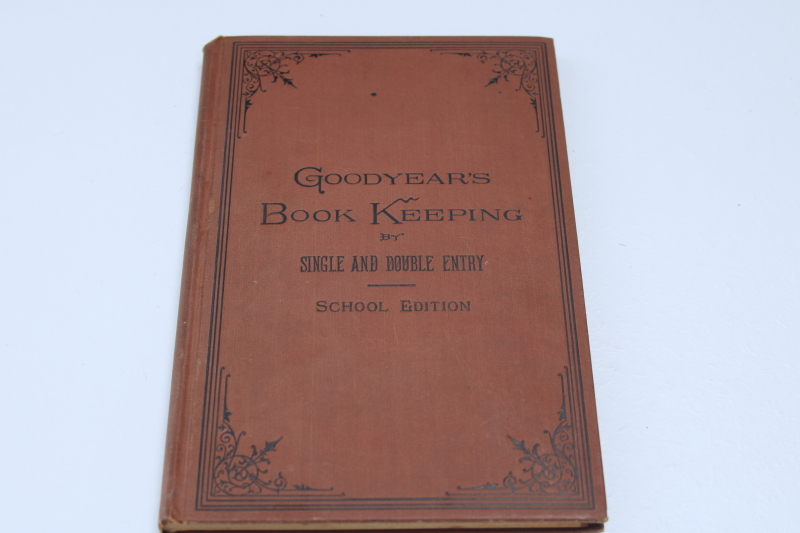This photograph showcases a well-worn, vintage book set against a light blue background. The book itself has a cover that appears to be a mix of burnt rust and brown hues, suggesting age and frequent use. The cover is bordered in an intricate black design, featuring a small arrow at the top and a circle at the bottom. The black lettering across the cover reads in a large, old-fashioned font: "Good Years Bookkeeping." Below this, in smaller font, it states, "Single and Double Entry." Following a thin horizontal line, it further specifies "School Edition" in all capital letters. The book gives off a distinctly antique vibe, with its cloth or leather-like cover adding to its historical allure. Photographed at a slight angle, the bottom of the book appears wider than the top, emphasizing its thinness and vintage charm. The background accentuates the book's aged character, making it the focal point of the image.